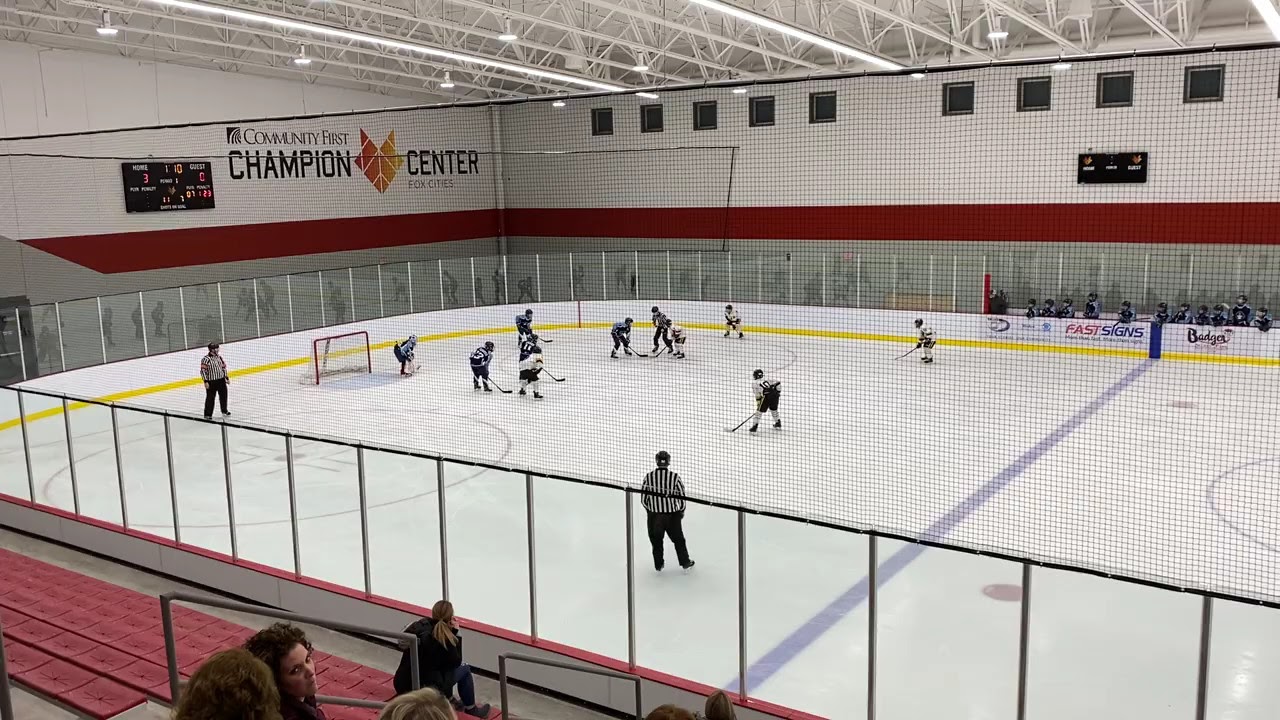This photograph captures a vibrant junior league hockey game taking place at the Community First Champion Center. The action is centered on a face-off, with two referees poised to drop the puck, and the young players, dressed in white or dark blue jerseys, are standing still, creating a moment of anticipation. The standard-sized rink is encircled by safety glass and netting, ensuring the crowd's protection. The arena is bathed in light from the white scaffolding overhead, with square windows near the roof letting in a bit of natural light. The scoreboard, partially obscured but showing a score of 3-0, is mounted on the left side of the rink. Spectators in red seats can be seen in the lower left-hand corner, while the opposing team watches intently from the bench on the right. The walls of the rink are white with bright yellow trim at the base, adorned with advertisement signs. Above the scoreboard, the name "Community First Champion Center" is prominently displayed, featuring a logo that resembles a leaf or a fox. The setting provides a dynamic yet organized view of a community-driven sporting event.